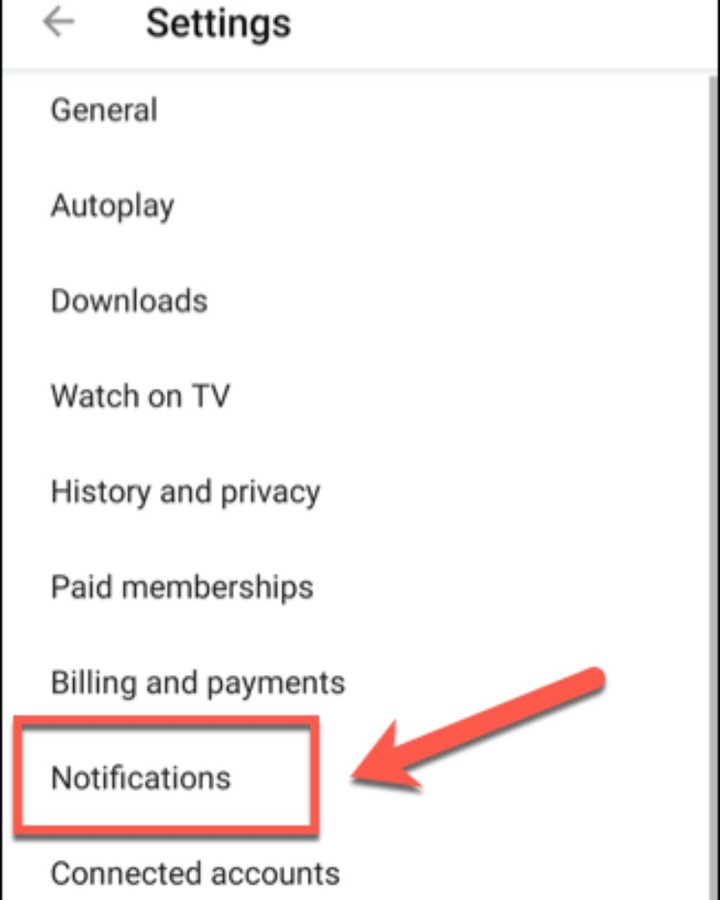The image displays a computer screen featuring a settings menu. At the top, the word "Settings" is prominently displayed in bold black lettering with a capital 'S', accompanied by a light gray arrow pointing to the left. Below the title, a vertical list of options is neatly arranged, each beginning with a capital letter followed by lowercase letters. The options listed include: General, Autoplay, Downloads, Watch on TV, History and Privacy, Paid Memberships, Billing and Payments, Notifications, and Connected Accounts. Each term is written in a plain charcoal-colored font. Highlighting the section, a red rectangle box surrounds the word "Notifications," and a large arrow directs attention towards this box. The screen also features two vertical black lines framing the sides, adding to the structured layout of the settings menu.